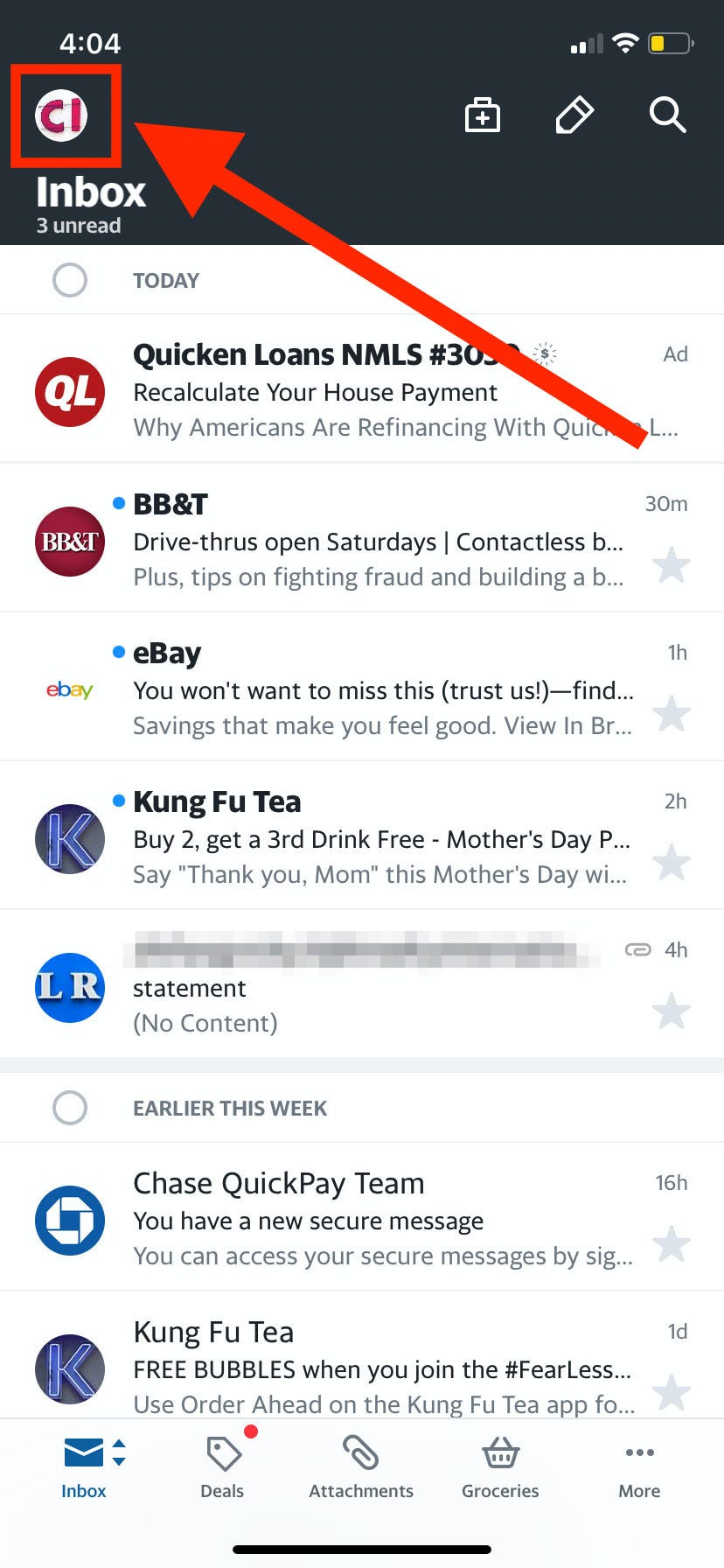**Caption**: This image resembles an inbox view on a mobile phone screen, featuring detailed elements and notifications. 

In the top left corner, the screen shows the number "404," while the top right displays icons for cellular signal, Wi-Fi, and battery status, which is yellow in this instance. Below, there's a conspicuous red "CI" in a white circle, highlighted by a large red arrow and a red box, likely edited in to draw attention to it. 

On the right side of the image, icons for a suitcase with a plus sign, a pencil, and a search magnifying glass are visible. The word "Inbox" appears below these icons, with the number "3" in red next to it indicating three new messages. Above "Inbox," the word "Today" indicates that these messages were received on the current day.

The first email, partially obscured by the red arrow, is from Quicken Loans, mentioning their NMLS number (partially cut off), and discusses recalculating house payments and reasons why Americans are refinancing with Quicken, trailed by an ellipsis.

The second email is from BB&T, concerning their open drive-thrus on Saturdays and offering contactless services, along with tips on fighting fraud and building something, ending with an ellipsis. This email was received 30 minutes ago.

The third email is from eBay, promoting savings deals with the subject "You won't want to miss this, trust us." The preview text continues with "savings that make you feel good," and ends with an ellipsis after "view in BR." This message was received one hour ago.

The fourth email is from Kung Fu Tea, advertising a “buy two, get a third free” promotion in honor of Mother’s Day. The message suggests saying thank you to mom with a special Mother's Day offer, ending with an ellipsis. This email was received two hours ago.